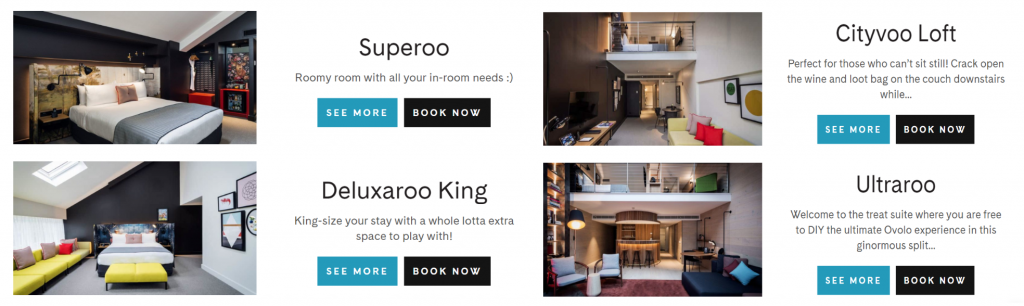This is a partial screenshot of a booking service website, potentially similar to Airbnb, displaying four room options with highly professional images and brief descriptions. The page layout appears incomplete, as it lacks the header and footer typically found on a full webpage. 

1. **Super Rule**: 
   - **Image**: Features a tastefully decorated bedroom in neutral tones like black, gray, white, beige, and brown.
   - **Description**: "Roomy room with all your in-room needs."
   - **Action Buttons**: "See More" and "Book Now."

2. **Deluxe Room King**: 
   - **Image**: A bedroom similar in design to the one above but with additional pops of color like yellow and red.
   - **Description**: "King-size your stay with a whole lot of extra space to play with."
   - **Action Buttons**: "See More" and "Book Now."

3. **City View Loft**: 
   - **Image**: Displays a loft with a living space, including a couch and a TV on the upper floor, decorated in mostly neutral colors with some yellow and red accents.
   - **Description** (truncated): "Perfect for those who can't sit still. Crack open the wine and loot bag on the couch downstairs while..."
   - **Action Buttons**: "See More" and "Book Now."

4. **Ultra Rule**: 
   - **Image**: The busiest of all images, showcasing a multi-level living area with a couch, shelving, lamp, bar stool, and a small wooden bar.
   - **Description** (truncated): "Welcome to the treat suite where you are free to DIY the ultimate overall experience in this ginormous split..."
   - **Action Buttons**: "See More" and "Book Now."

Each room option is visually appealing with descriptions aimed at enticing potential guests, further complemented by actionable buttons for more details or reservation.